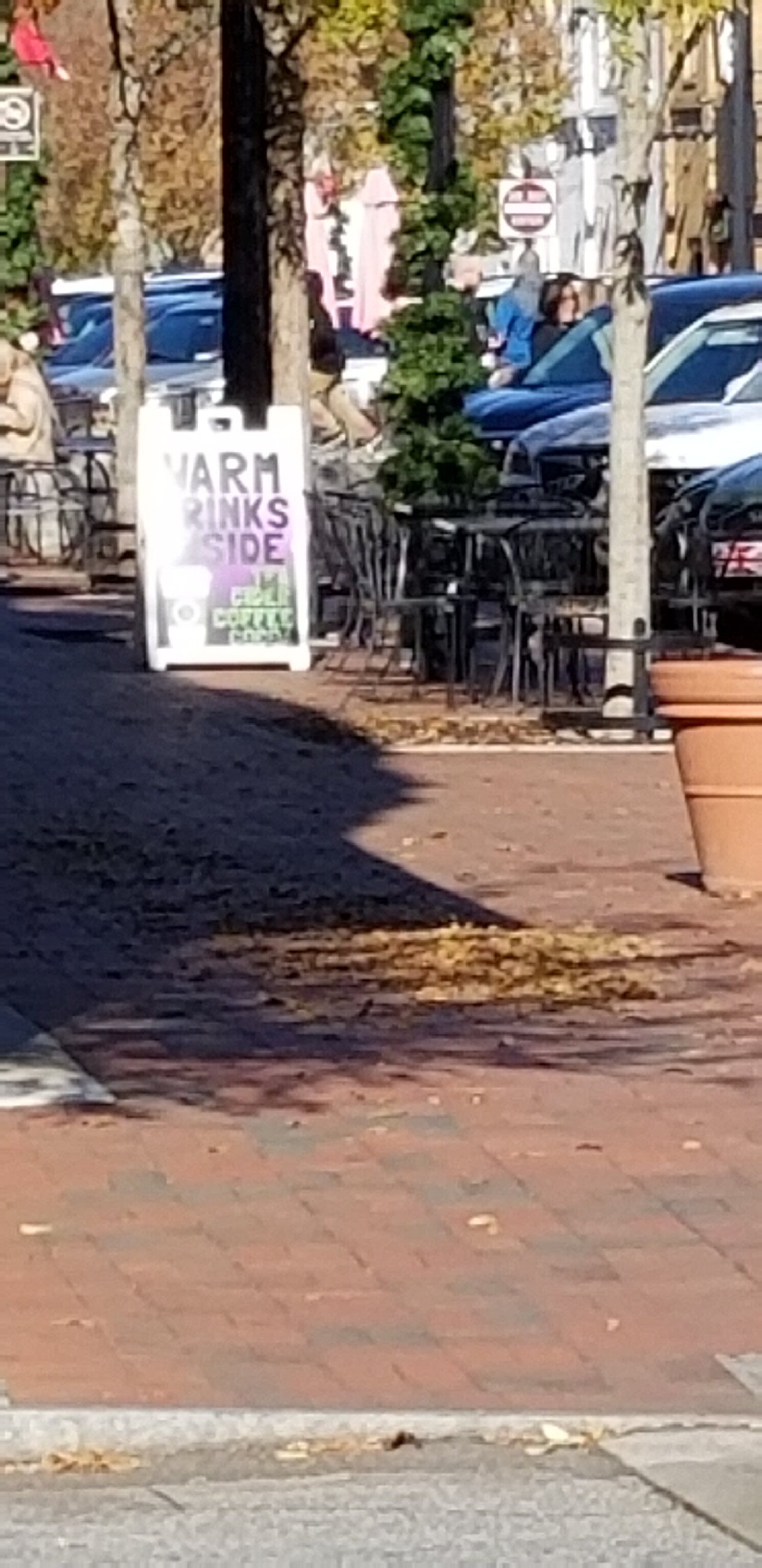The image captures a picturesque street scene featuring a red brick sidewalk in front of various businesses, which gives a charming and quaint feel reminiscent of an outdoor street cafe. The sidewalk, partially covered by brownish fallen leaves, abuts the edge of a road that is visible at the bottom of the photo. On the right side, a large terracotta planter adds a touch of greenery and warmth. Nearby, several black metal cafe tables and chairs invite passersby to sit and enjoy the ambiance. A small, white folded sign with blue letters, displaying "warm drinks inside" and an image of a coffee cup, sits on the walkway, hinting at a cozy coffee shop just steps away. The left side of the sidewalk is shaded by the building, casting cool shadows on the ground. Trees line the street, with cars parked in parallel spaces and a 'do not park' sign visible across the street in the background. Additionally, little fences surround the base of the trees, adding to the organized and well-kept appearance of the area.